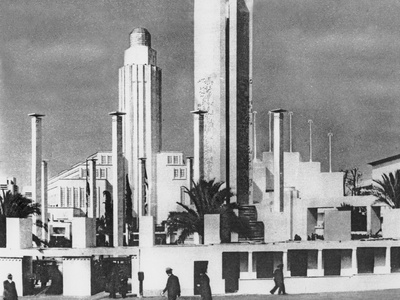This is a small, grainy black-and-white image depicting a highly detailed, futuristic cityscape with elements of Art Deco architecture. Prominently, there are two main structures in the background: a shorter cylindrical tower on the left and a very tall, rectangular skyscraper on the right. Surrounding these towers are smaller white buildings that appear to lack windows, enhancing the modern aesthetic. Streetlights resembling stone pillars with small lamps on top are evenly spaced across the scene. 

In the foreground, there's a rectangular archway at street level, framed by a sidewalk bustling with people dressed in black suits and hats. They seem to be walking in and out of entrances that resemble underground garages or passageways through a wall adorned with Art Deco features. Additionally, there are palm trees and plants with long leaves lining this wall, adding a touch of greenery to the otherwise monochromatic and architectural landscape. The sky overhead appears overcast, contributing to the overall dramatic and somewhat surreal atmosphere of the city.